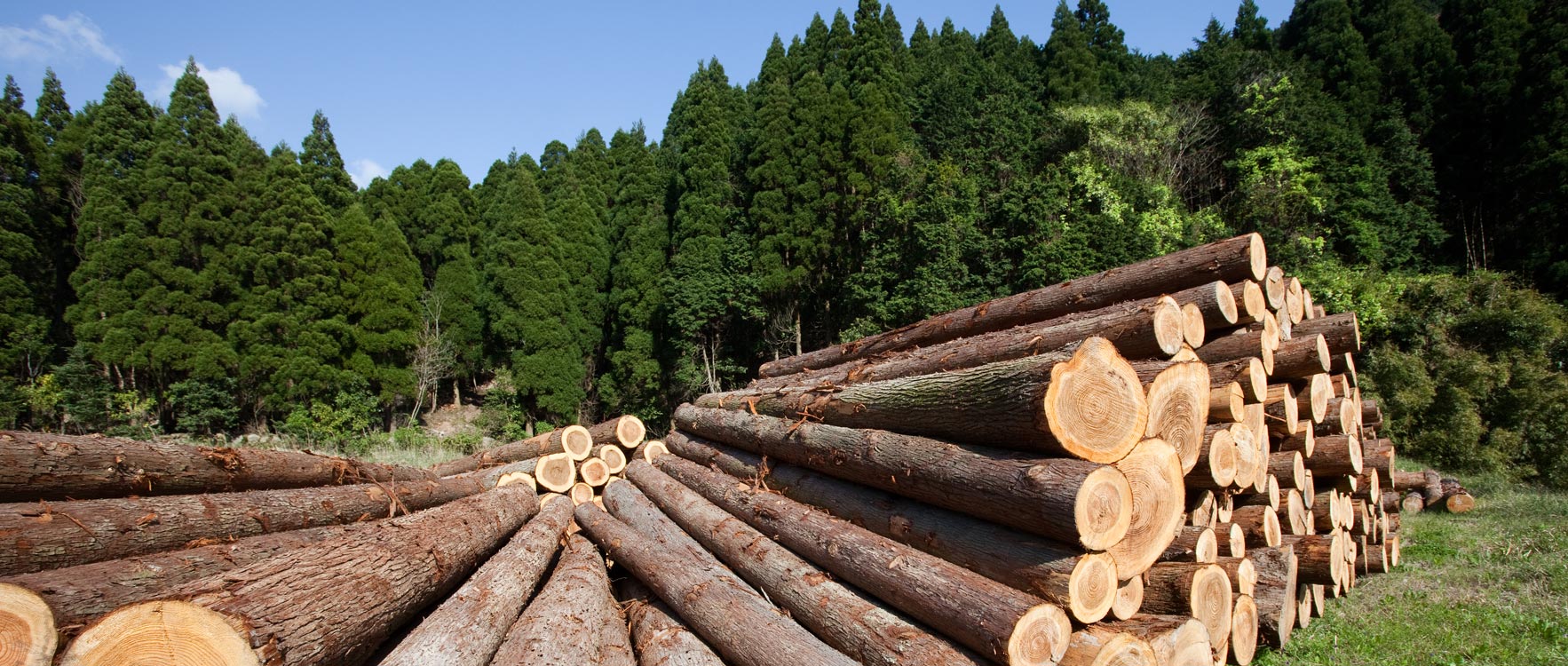The image depicts a bright, sunny day at an outdoor lumberyard, set against a clear blue sky with a few white clouds and the sun shining through. In the foreground, there is a field of vibrant green grass, where multiple logs lie stacked atop one another. These logs, dark brown on the outside and light beige on the inside, have been cut from the dense forest seen in the background. The forest is composed of medium-height trees, likely evergreen, with a refreshing shade of bright green leaves, creating a rich, natural backdrop. Some small knobs are visible on the sides of the logs. Another pile of logs can be seen behind the first, reinforcing the industrious atmosphere of the lumberyard. The overall scene is expansive, captured in an ultrawide shot that immerses the viewer in this tranquil yet industrious woodland setting.